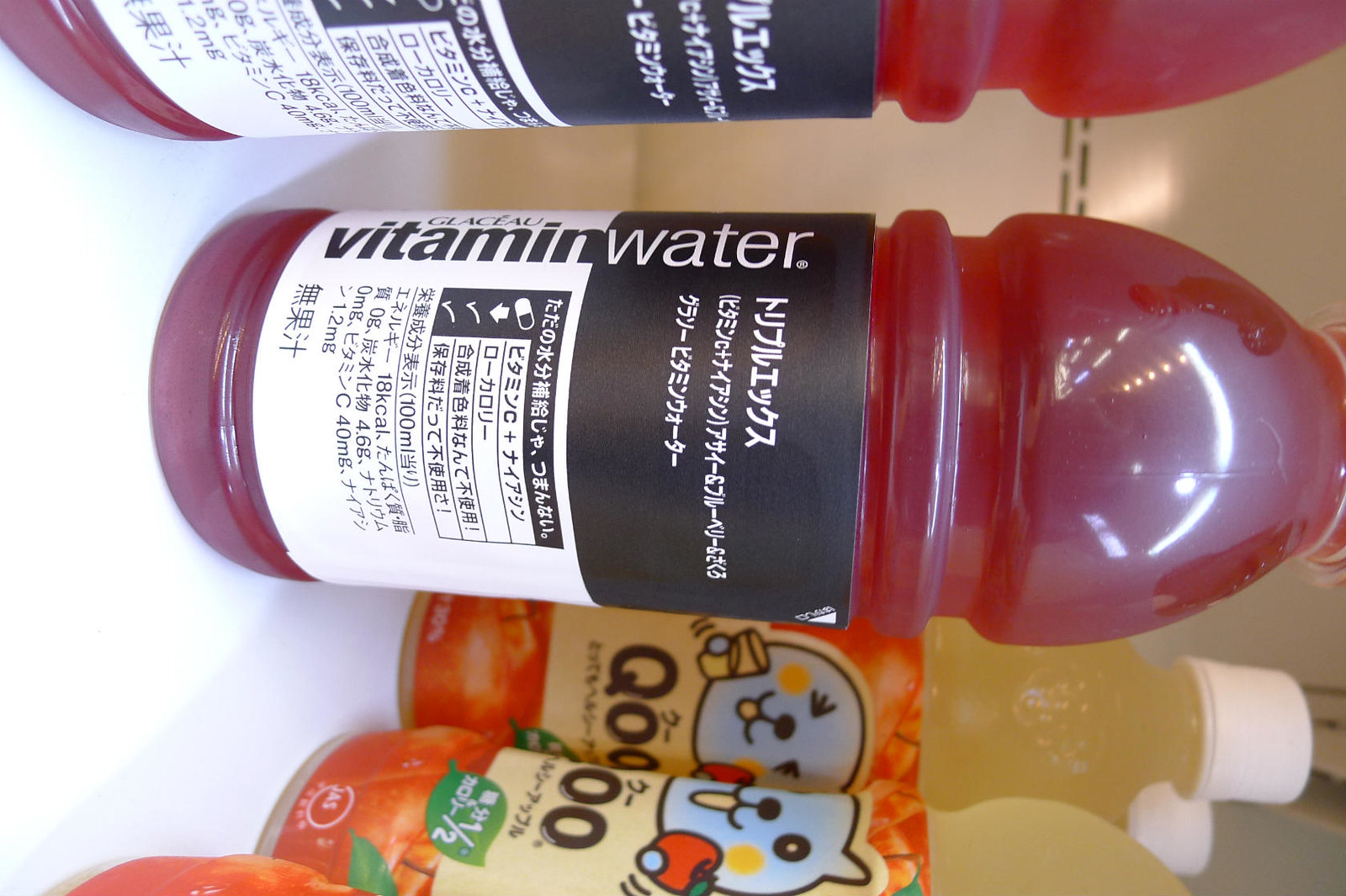This photograph, currently displayed sideways and needing a 90-degree counterclockwise rotation to be viewed correctly, features an assortment of drinks bottles. Central to the image is a bottle of Vitamin Water filled with a dark red, fruit punch-like liquid. This bottle's labeling is noteworthy: the top half of the label is black with white writing, and the bottom half is white with black writing, featuring text in Japanese, particularly katakana symbols. To the left of this bottle, partially out of the frame, is another identical bottle of Vitamin Water. On the right side of the image sits a distinct bottle, possibly containing apple juice. It has an orange hue and a white cap, with a label depicting a blue, animated circular face, possibly a cat, holding a glass. This bottle is branded with the characters "QOO," and images of apples can be seen near its base. Overall, there are four to five bottles visible, with two clearly identifiable as Vitamin Water and the others being less discernible.